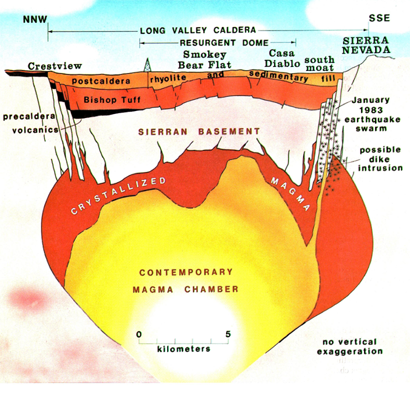This detailed cross-section diagram of the Long Valley caldera reveals multiple geological layers and features associated with volcanic activity. The top of the image shows labels such as "Chris View," "Smoky Bear Flat," "Casa Diablo," "South Moat," and "Sierra Nevada," overlaying a blue sky. Beneath this, the surface layer is marked as "Postcard Caldera" composed of "Rhyolite" and "Sedimentary Fill." Below this layer, a darker red strata is labeled "Bishop Tuff," which transitions into a white rocky layer designated as the "Sierran Basement." Further down, there is a red layer identified as "Crystallized Magma," and at the bottom, a large yellow area represents the "Contemporary Magma Chamber." Notable demarcations include a marked earthquake occurrence in 1983 and indications of a possible dike intrusion. The diagram includes a scale indicating a span from zero to five kilometers, highlighting the vastness of the volcanic structures. This visual is enriched with notes and geological terminologies, presenting a comprehensive look at the inner workings of a caldera.